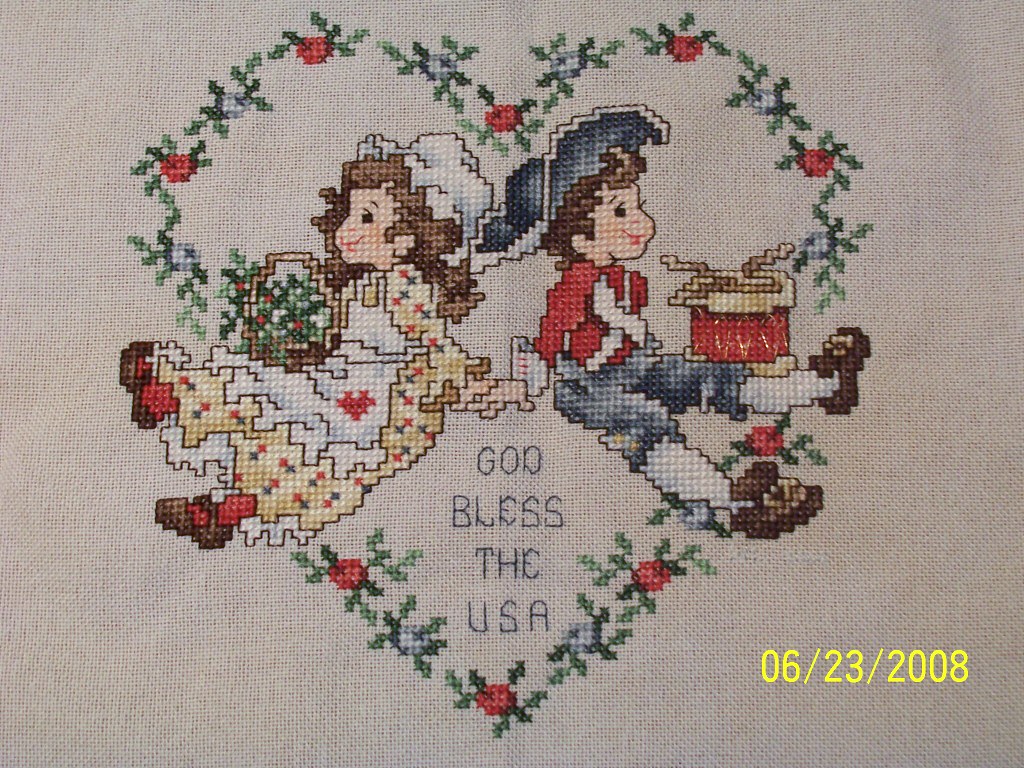This cross-stitch design, evocative of a tapestry, features a heart-shaped arrangement of red roses and green leaves against a light gray background. At its center, two illustrated children in traditional colonial attire sit back-to-back, holding hands. The boy, positioned on the right, dons a blue tricorner hat and holds a red drum with drumsticks. The girl, on the left, wears a long floral dress with an apron and a white bonnet, holding a basket of flowers in her lap. Above them, in blue stitching, appears the phrase "God Bless the USA." The detailed embroidery captures the charm and innocence of the scene, marked with a timestamp indicating it was completed on June 26, 2008.